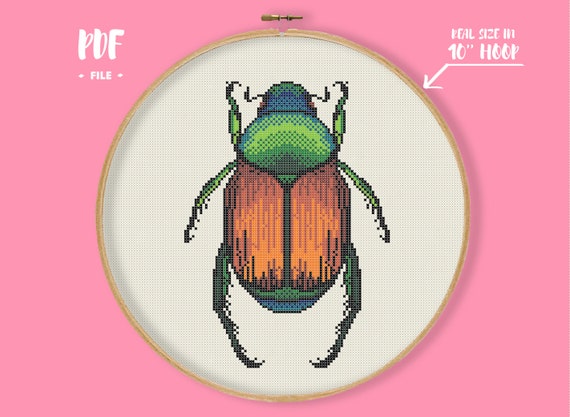The image showcases a detailed diagram likely intended for a cross-stitch pattern. Dominating the image is a large rectangular format with a bright pink background. On the top left, in white text, "PDF file" is prominently displayed. On the top right, also in white text, there's an indication of "real size in 10 inch hoop" with an arrow pointing towards the center. At the center of the image is an embroidery hoop made of wood, containing a completed cross-stitch project of a beetle. The beetle is depicted with a primarily green body, featuring jade tones, complemented by bronze or copper-colored wings, six legs, and two antennas. The hoop and its contents cast a slight drop shadow against the pink background. This imagery, possibly meant for a listing, indicates that the cross-stitch project could either be a pattern for a PDF purchase or a fully finished piece available for purchase. The rectangular image is slightly more squat in shape compared to a traditional flag.